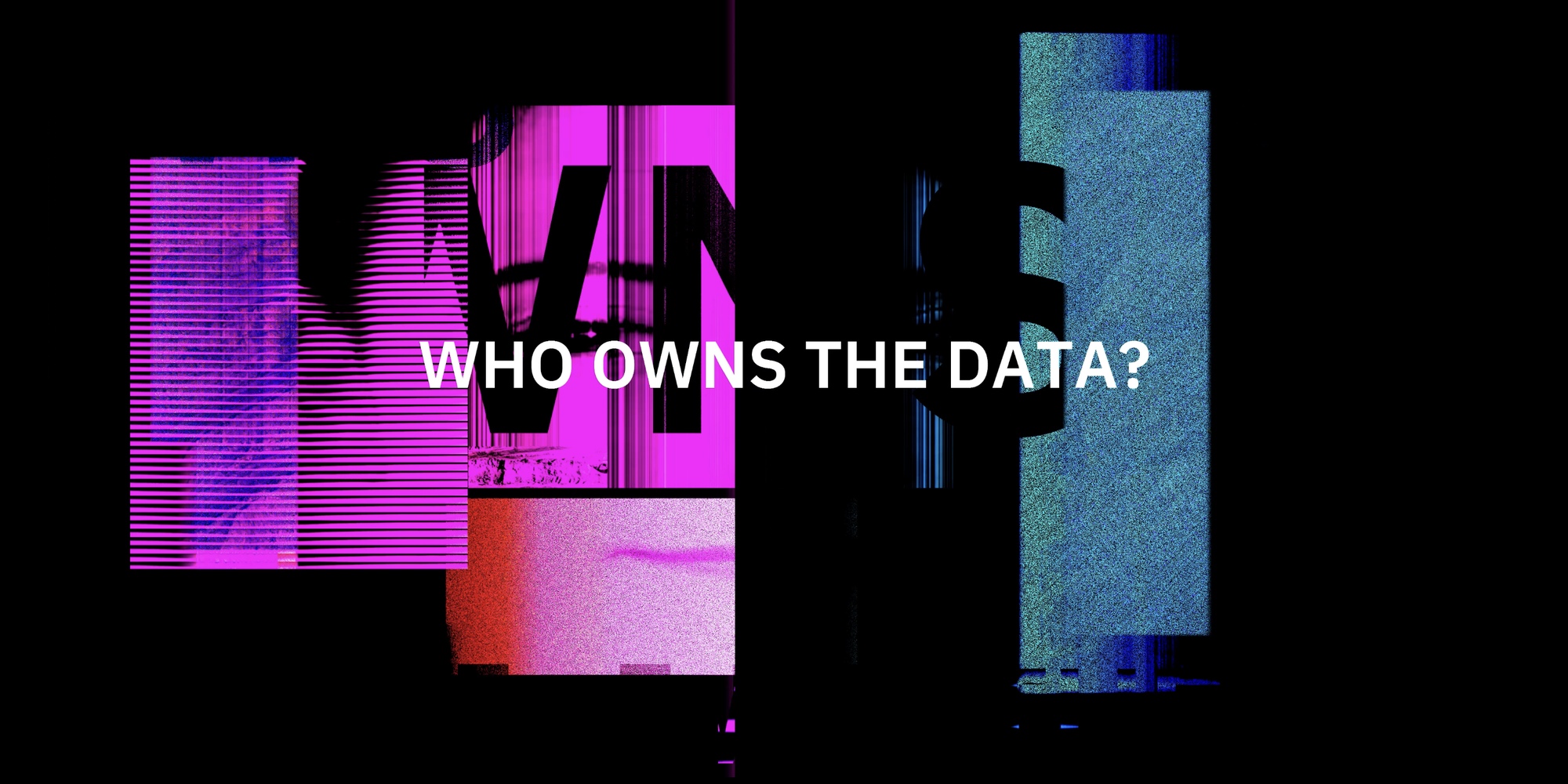The image features a jet-black rectangular background with an assortment of vibrant and complex visual elements layered on top. Dominating the center is bold white text that reads "WHO OWNS THE DATA?" in all caps. Surrounding this text is an eclectic mix of rectangles and bars in shades of light blue, deep blue, hot pink, and purple, interspersed with abstract designs and static patterns reminiscent of a television losing signal. Notably, there are fragmented images of a woman’s face – her eye and eyebrow in one vibrant purple rectangle, and a portion of her lips in another lighter purple box with an orangish hue. Additional elements include narrow vertical stripes of hot pink and dark blue rectangles stacked on top of each other, contributing to a chaotic yet cohesive digital collage. The intricacies and the color palette suggest that the image might be a slide from a presentation or a piece of graphic design pulled from a website. Faint, indecipherable letters and imprints in the background add an extra layer of texture and depth to this visually engaging composition.